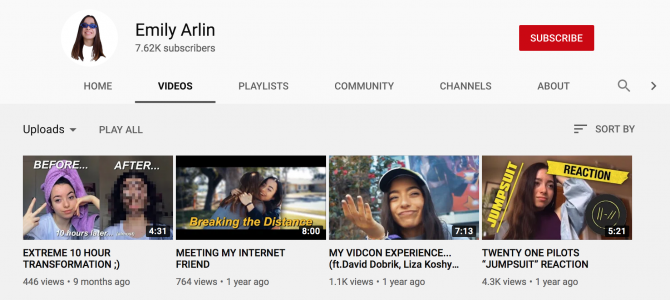This is Emily Arlen's YouTube channel page, featuring a sleek white background with gray text at the top. Emily Arlen, who has 7.62k subscribers, is depicted in the profile picture as a woman with brown hair wearing sunglasses and a white shirt. Adjacent to the profile picture, a red button labeled "Subscribe" is prominently displayed. The navigation menu includes options such as "Home," "Videos" (highlighted in black), "Playlists," "Community," "Channels," and "About." A magnifying glass icon and an arrow symbol are also visible for search and navigation purposes.

Scrolling down, the "Uploads" section is highlighted with an arrow and "Play All" button alongside it. On the right, there's a "Sort by" option with corresponding lines. 

In the list of video thumbnails:

1. The first video features a split image labeled "Before" and "After." On the left, Emily is shown with a purple towel on her head and a white shirt, holding up some fingers. The "After" side is blurred. This video, titled "Extreme 10 Hour Transformation," is 4 minutes and 31 seconds long, with 446 views from nine months ago.

2. The second video thumbnail shows Emily hugging another woman and is titled "Gold Bottom Breaking the Distance," with the subtitle "Meeting My Internet Friends." It is 8 minutes long, with 764 views from one year ago.

3. The third video, "My Viking Experience Featuring David Dobrik and Liza Koshy," is 7 minutes and 13 seconds long. The thumbnail shows Emily wearing a baseball cap with her hand outstretched and flowers in the background. This video has 1.1k views from one year ago.

4. The last video thumbnail displays Emily looking off to the side in grayscale attire. Titled "21 Pilots Jumpsuit Reaction," this 5-minute and 21-second video has amassed 4.3k views from one year ago.